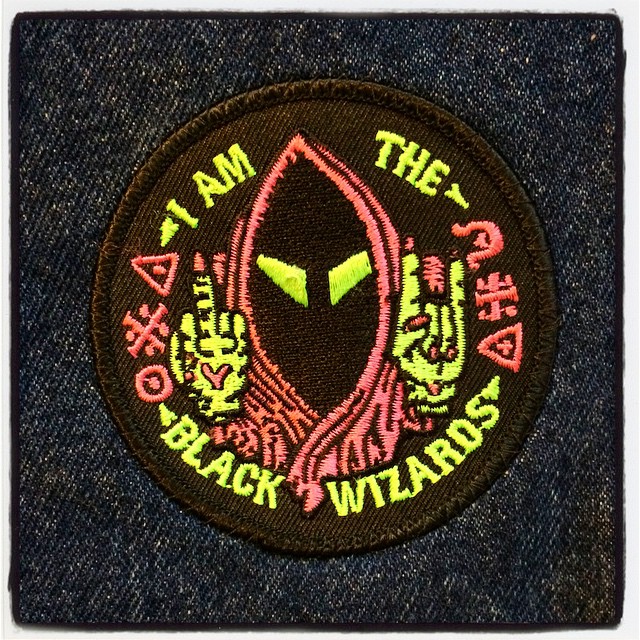This image depicts a close-up of a black circular embroidered patch affixed to dark blue denim, likely part of a jacket or vest. The patch features a hooded, druid-like figure with a faceless, black interior except for two large, rectangular glowing yellow-green eyes. The character is clad in a pinkish-reddish hood and has green hands, one making a middle finger gesture and the other forming a hang loose or devil horns sign, with pink nail polish visible. In neon yellow text, the patch reads "I Am The" at the top and "Black Wizards" at the bottom. This text refers to a song by the black metal band Emperor, entitled "I Am the Black Wizards." The design is surrounded by various symbols, including triangles and dots, giving the patch a mystical aesthetic. The luminescent neon colors, mainly pink, yellow, and green, add vibrancy to the detailed design, making it a distinctive emblem for fans of the band or those perhaps belonging to a fictional "Black Wizard Club."